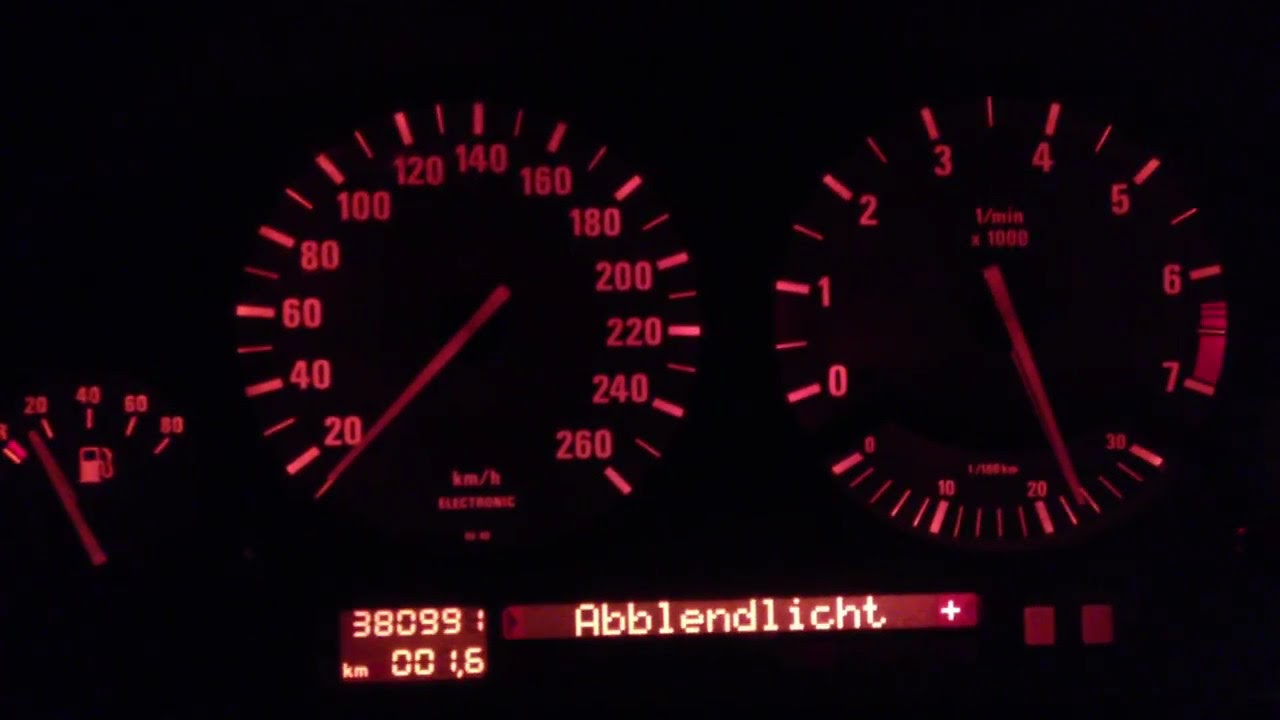The image shows a digital automobile dashboard photographed at night, with a pitch-black background illuminated solely by red lights and text. Dominating the center are two large gauges. The left gauge is a speedometer marked in kilometers per hour, ranging from 20 to 260 KPH, with a prominent red needle. Adjacent to it on the right is a tachometer, displaying values from 0 to 7. Further to the left, there is a fuel gauge. In the bottom middle of the image, an LCD screen displays various readings. The left part of the screen shows the car's mileage of 380,991 kilometers, while the center of the screen features the German word "Ablendlicht" and a plus sign. Below the main gauges, there are additional smaller rectangular indicators displaying numbers and text, all illuminated in the same distinct red hue. The entire scene is set against a starkly contrasting black background, highlighting the illuminated elements of the dashboard.